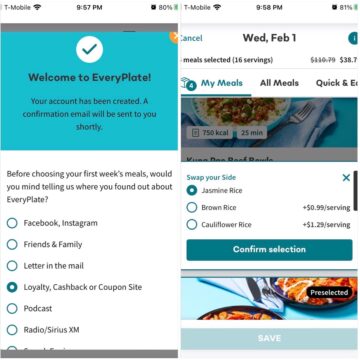The image consists of two phone screenshots displayed side-by-side:

**Left Screenshot:**
- The top background is greyish, displaying "T-Mobile" in black along with a blurry Wi-Fi signal indicator. The time is shown as either 8:57 PM or 9:57 PM with the battery at 80% charge.
- Beneath the top border, there’s a grey divider line followed by a teal background.
- In black text, there’s a message: "Welcome to EviePlay. Your account has been created. A confirmation email will be sent to you shortly."
- There’s a white circle with a teal checkmark inside it.
- An orange circle with a white "X" is partially visible, indicating additional information or options cut off from view.
- Below this, there’s a question: "Before choosing your first week's dinner, would you mind telling us where you found out about EviePlay?"
- The user selected "Loyalty cashback or coupon site" from several options, which include "Facebook," "Instagram," "Friends/Family," "Letter in the mail," "Podcast," and "Radio/Sirius XM."

**Right Screenshot:**
- The header similarly shows "T-Mobile" with a time of 8:58 PM, just one minute after the first screenshot. The battery now displays a charge of 81%.
- Below, there’s a teal bar with the option "Cancel" in black text. It indicates the date as "WED February 1st" and "Black male selected," possibly referencing a user's profile.
- It shows information about servings, mentioning "16 servings" without price details. A fragment mentions "The fresh number by juicy 38.7," though it’s cut off.
- In teal text, it says "My Meals," followed by "All Meals" and "Quick and Easy," though the latter is cut off.
- An image of a plate of pasta with broccoli is visible, labeled "750 KCL" and a preparation time of "25 minutes."
- Below this, it gives options for swapping the side dish. "Jasmine Rice" is selected, with other choices being "Brown Rice" (99¢ extra per serving) and "Cauliflower Rice" ($1.29 extra per serving).
- There’s a teal rectangular box with "Confirm Selection" in white text.